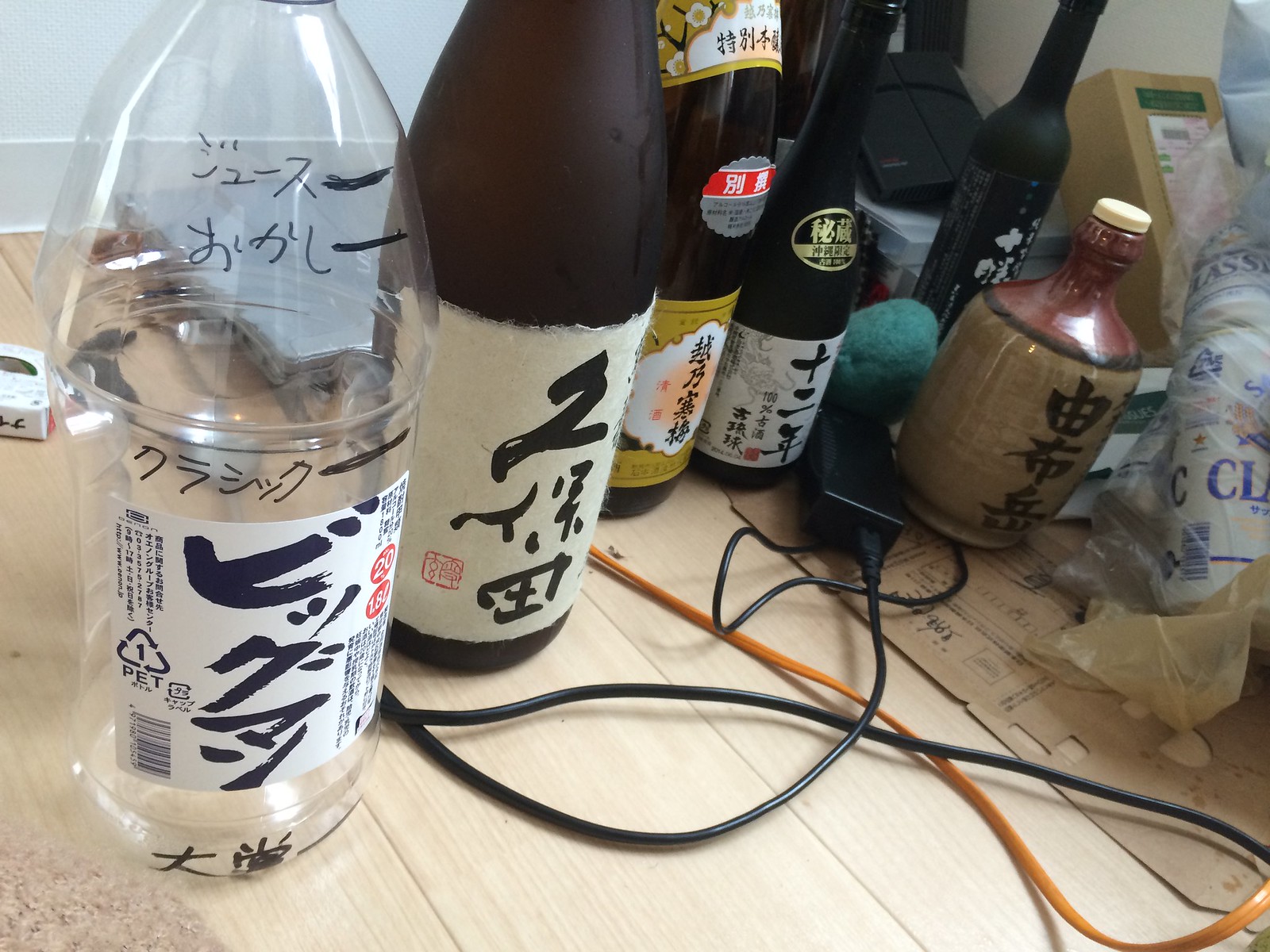The image depicts a close-up of a cluttered floor made of light wood grain, featuring a diverse collection of at least five Japanese alcoholic drink bottles in various shapes and sizes. Starting from the left, a clear empty bottle with a white label and additional black marker writing stands out. Next to it, there's a matte black bottle with remnants of a torn-off white label bearing black lettering. Moving right, two brown glass bottles are visible, one with a yellow label and the other with a white label, both displaying black lettering. Further right, a distinctive jug with a brownish-red top and a tan body, adorned with black Asian characters, sits amidst the items. On the far right, two beer cans are encased in a clear plastic bag. The backdrop includes a mix of scattered items like wires, possibly a laptop charger, and a small laptop behind the clear plastic container, adding to the scene's clutter. A white wall with woodwork frames the chaotic arrangement, emphasizing the various textures and elements present in this detailed snapshot.